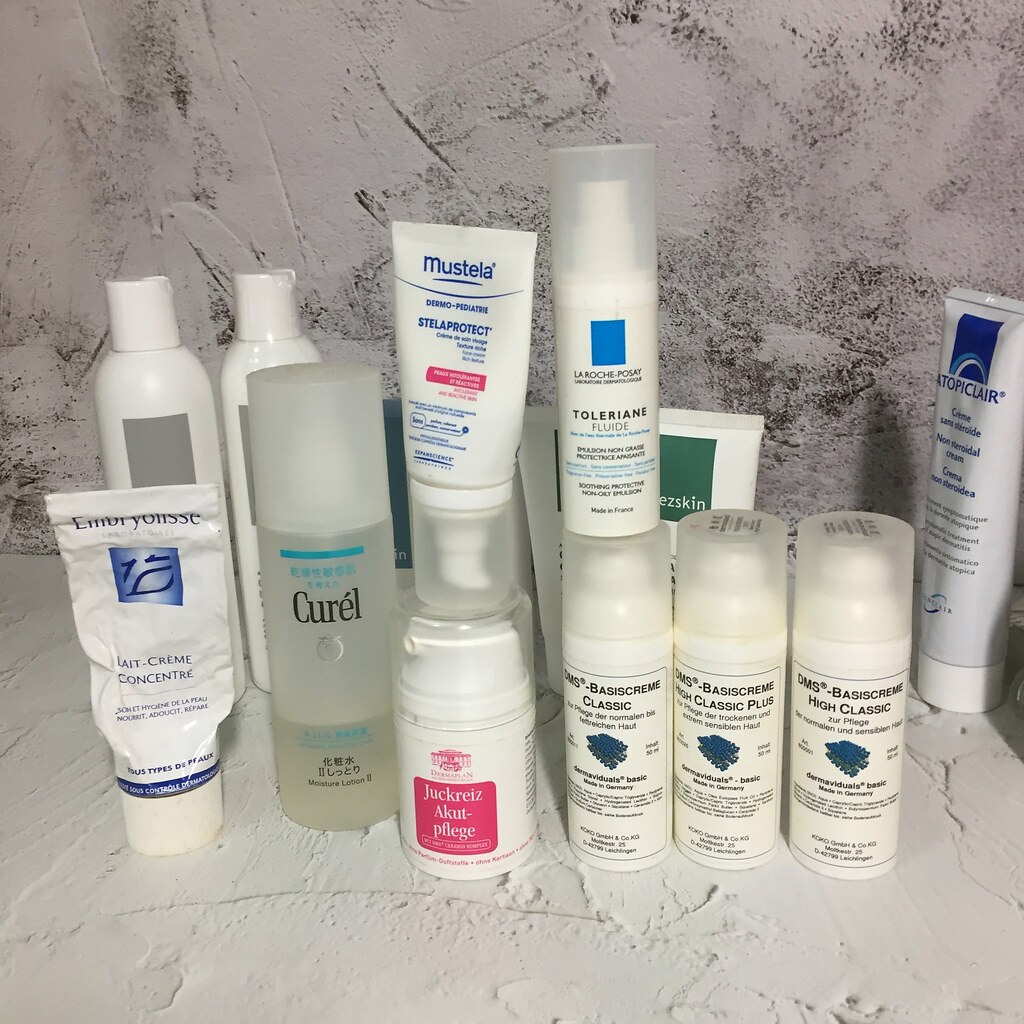The photograph showcases an arrangement of various skincare products placed on a rough, unevenly painted white surface, reflecting signs of wear from multiple paint layers. Behind the items, the wall is similarly aged, with white paint revealing brown undertones where it has worn away. 

On the left side of the image, there is a white tube of Embryolisse Lait-Crème Concentré. Beside it stands a frosted clear bottle labeled Curel. Next in line is a white pump bottle with a pink label that reads Jacre's Acute Fledge, topped with the word Dermaplan. Resting atop this bottle is another pump tube labeled Mustela, Stella Protect. 

Further to the right, there are three identical bottles labeled DMS Basis Cream Classic, featuring white bodies and frosted clear tops. Atop one of these bottles rests a bottle of La Roche-Posay Toleriane Fluid. 

In the background, several other bottles are partly obscured. To the left, two tall white bottles with gray labels are partially hidden behind the front row. A tube with a green label marked Easy Skin is visible as well. On the right side of the composition, there is a white tube with a white top labeled Atopiclair. 

The cluttered arrangement and the weathered backdrop add a sense of authenticity and use to the collection of skincare products.